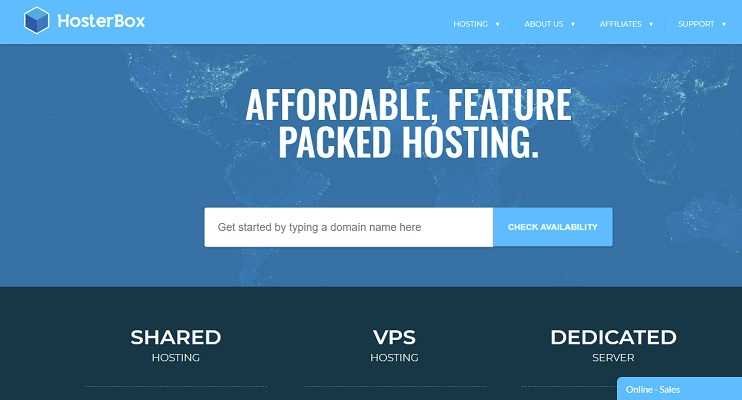**Header:** A light blue header tops the image, set against a blue background, creating a visually pleasing and cohesive design. 

**Main Content:** The main section of the image features a centrally located white box. Dominating this space is a prompt that reads, "Get started by typing a domain name here," inviting users to engage directly. Beneath this text is a blue rectangular button, clearly labeled with the words "Check Availability" in white, to facilitate the next action step seamlessly. 

**Footer:** The footer is rendered in dark blue, contrasting with the header and main content, to neatly close off the design. Within the footer, several hosting options are prominently displayed:

- **Shared Hosting:** The word "Shared" is in a larger, bold font, emphasizing its importance.
- **VPS Hosting:** Here, "VPS" is capitalized, larger, and bolded, ensuring it stands out more than the word "hosting."
- **Dedicated Server:** Similarly, "Dedicated" is in a larger, bold font compared to "server," highlighting its significance.

**Additional Elements:** In the bottom right corner of the footer, a blue rectangle catches the eye with the words "Online Sales" written in white, directing users to this section for more information or to initiate purchases. 

**Brand Elements:** Integrated into the design is the "hoster box," a white box featuring a blue cube, symbolizing the brand. This box also includes sections titled "Hosting," "About Us," "Affiliate," and "Support," each likely leading to further details about the services provided.

Overall, the image successfully combines various visual elements and text formats to guide the user through the information and actions effectively.